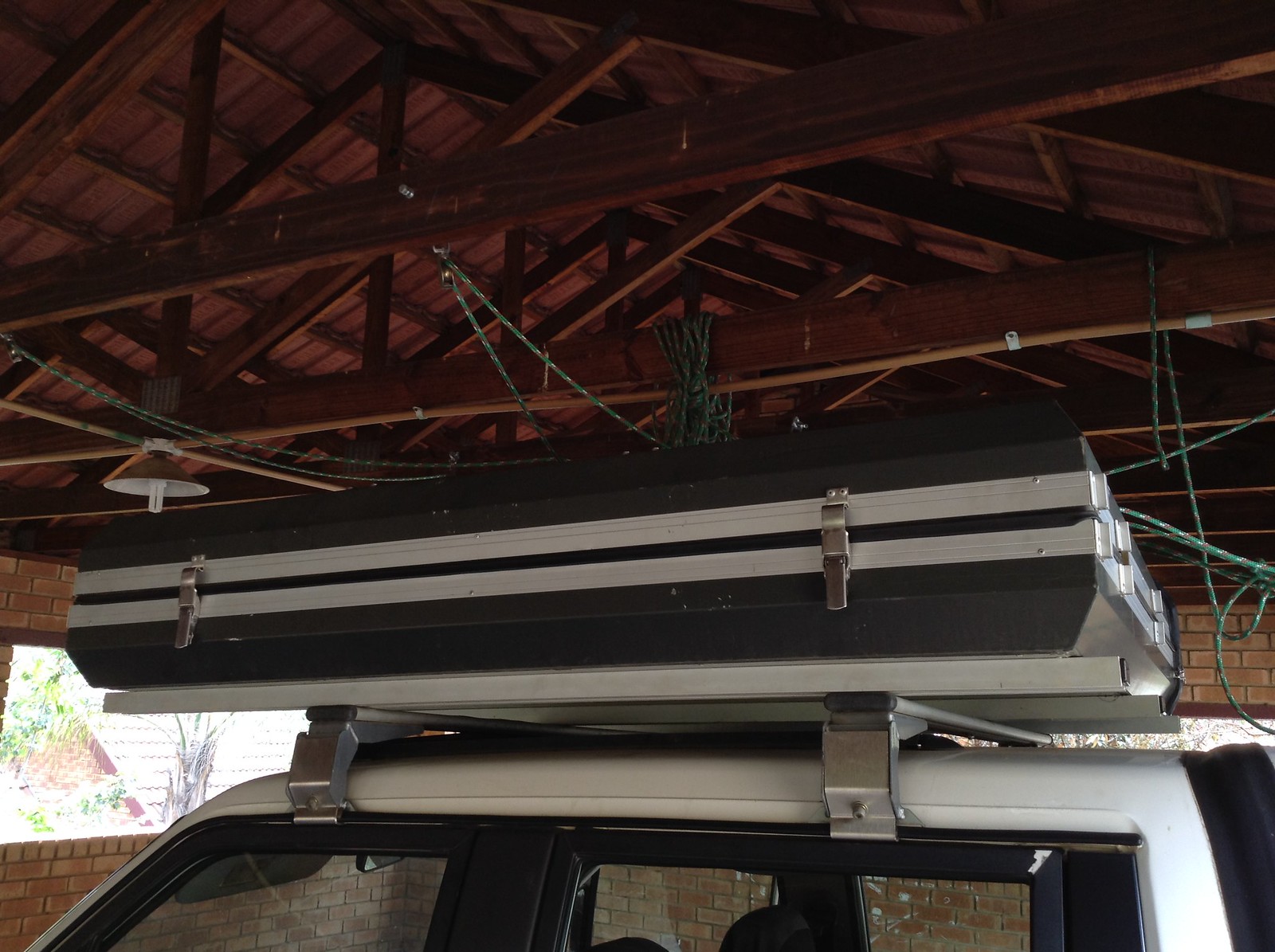The image captures a white SUV-like vehicle parked inside a partially open garage with brick walls. The garage features vaulted wooden ceilings, revealing visible struts and support beams entwined with green nylon ropes. Atop the vehicle is a large black case secured with metal clamps and bearings. This case spans the width of the vehicle and has silver accents along the top and bottom, and is clamped shut with two silver latches, suggesting a vertical opening. The ambient daylight filters through the open-air windows, offering glimpses of an outside environment with trees and possibly a house. A ceiling light fixture is present but remains unlit.